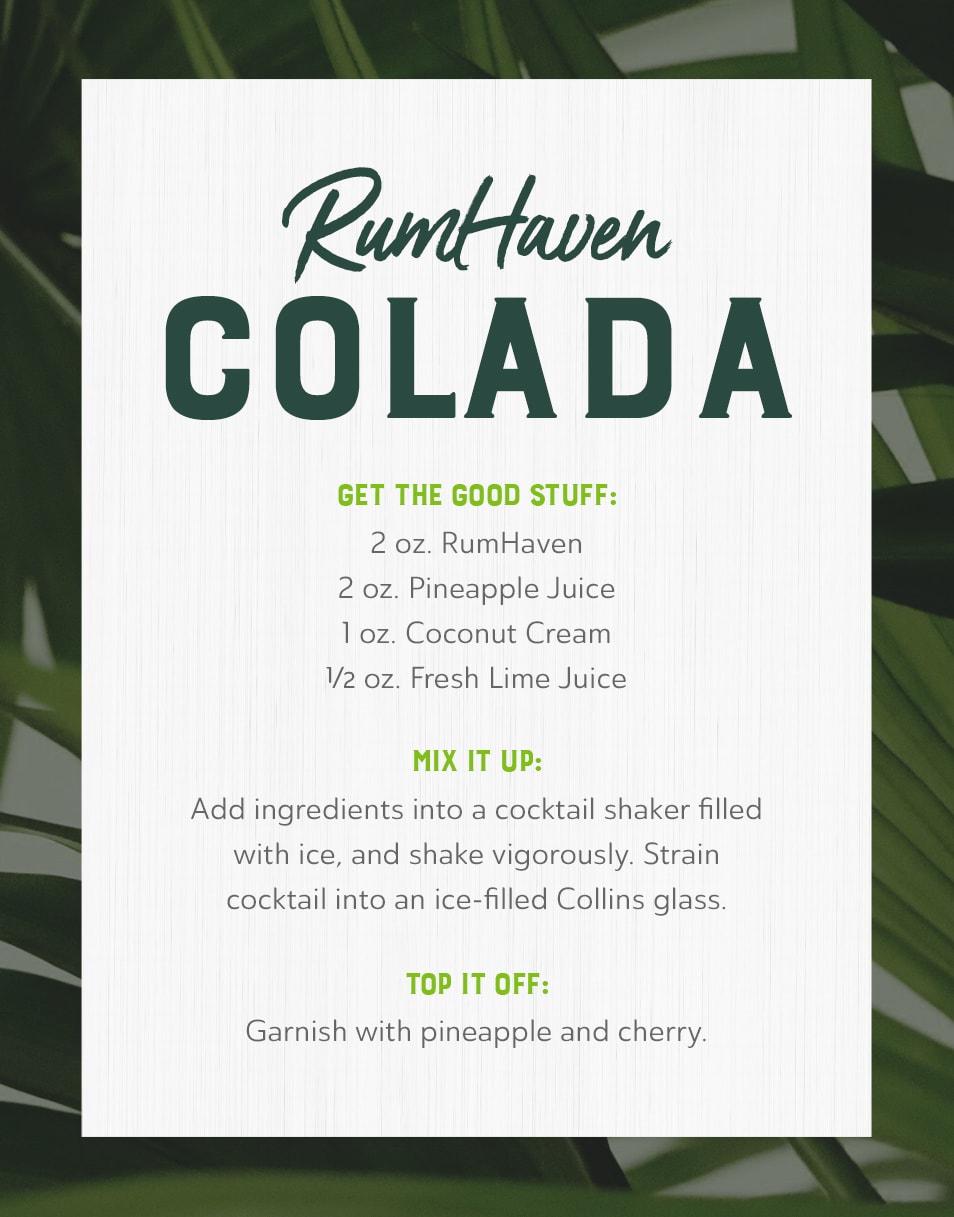The image displays a detailed recipe for a cocktail drink named the Rumhaven Colada. The recipe is presented on a white rectangular card that features subtle textured lines and is surrounded by a thick border of palm fronds in light greens and whites. At the top of the card, prominently centered in large green text, is the title "Rumhaven Colada." Below this, in smaller green text, is the phrase "Get the good stuff." The list of ingredients follows in black text: 2 ounces Rumhaven, 2 ounces pineapple juice, 1 ounce coconut cream, and 1/2 ounce fresh lime juice. Moving further down, the card in green text advises to "Mix it up," and the black text instructs to "Add ingredients into a cocktail shaker filled with ice and shake vigorously. Strain cocktail into an ice-filled Collins glass." Toward the bottom, the card in green text says "Top it off," and in black text finishes with "Garnish with pineapple and cherry." The design features a harmonizing palette of greens and whites that underscore the tropical theme of the cocktail.